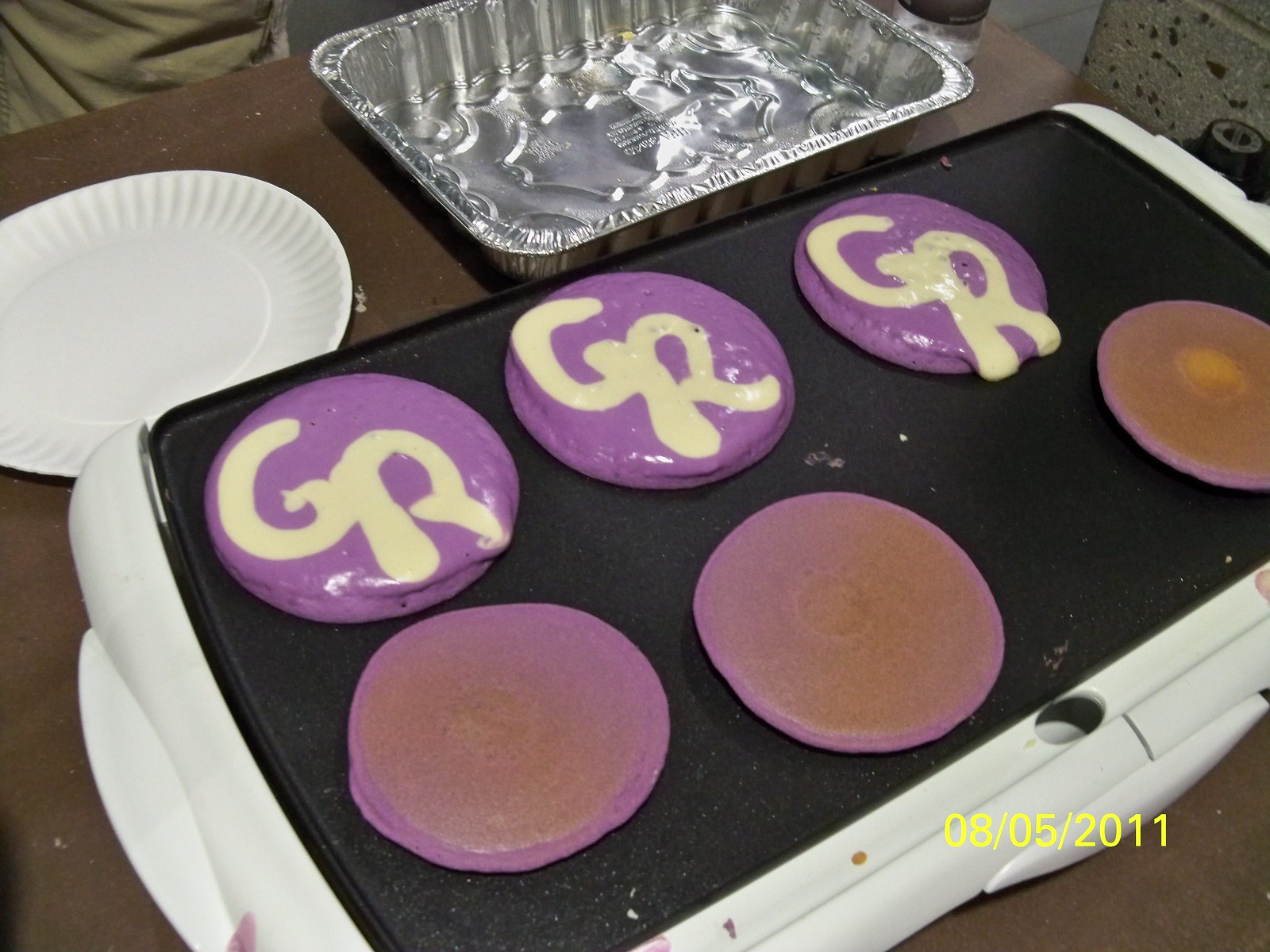The image features a close-up view of a white-edged, black-surfaced griddle holding six decorative pancakes. The griddle, equipped with two small drawers for catching droppings, rests on a brown table. Three pancakes at the bottom have already been flipped, while the three on top showcase a purple frosting adorned with white letters 'G' and 'R'. The batter for all the pancakes has been dyed purple. In the lower right corner of the image, the date "08/05/2011" is displayed in yellow. Accompanying the griddle on the right is an aluminum pan, and to the left, a white paper plate. The edge of a clear glass bottle with a black label is also partially visible near the arrangement.